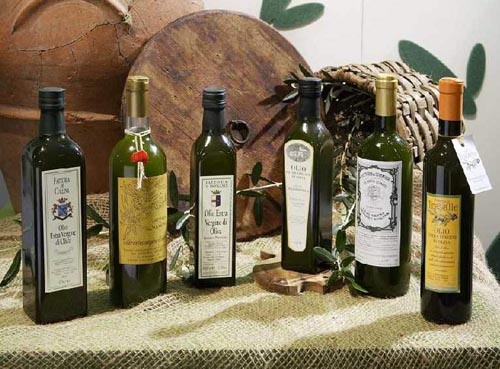This indoor photograph displays a collection of six bottles, possibly olive oil or wine, arranged on a table draped with a greenish-yellow cloth. The background features a white wall decorated with cut-out dark green leaves and round wooden barrel lids with holes at their centers. There's also a wicker basket tipped on its end, revealing its light brown texture.

From left to right, the bottles vary in color and shape:
1. The first bottle is black with a black cap and a white label.
2. The second is a green cylindrical bottle with a gold cap, adorned with a white string and a small red flower, and it has a yellow label.
3. The third bottle is black and thin with a white label and a black cap.
4. The fourth bottle, similar to the third, is also black with a white label and black cap.
5. The fifth bottle is dark green, cylindrical with a gold cap, and features a white label with a black border.
6. The last one, on the right, is cylindrical with a light brown cap and a yellow label. It also has a white rectangular tag, possibly a price tag.

Behind the bottles, on the wall, there's an array of large cylindrical wine holders and, to the right, a dark brown lid. The scene is further embellished with leaves and branches that extend from behind the bottles, adding a natural touch to the arrangement.